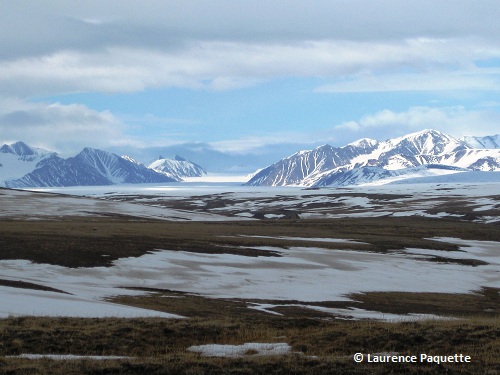This vibrant landscape features a stunning mountain range cloaked in snow, reminiscent of a hand-tinted postcard. The snow-capped peaks glisten under faint sunlight, reflecting off the crisp, icy surfaces. Above, the sky is a soft blue adorned with layers of grayish and whiter clouds, adding depth to the serene atmosphere. In the foreground, low, snow-dusted hills and patches of brown grass provide contrast to the pristine white of the mountains, creating a textured, almost painting-like effect. The scene is embossed with the name "Lawrence Paquette" in the bottom right corner, indicating the photographer's copyright.